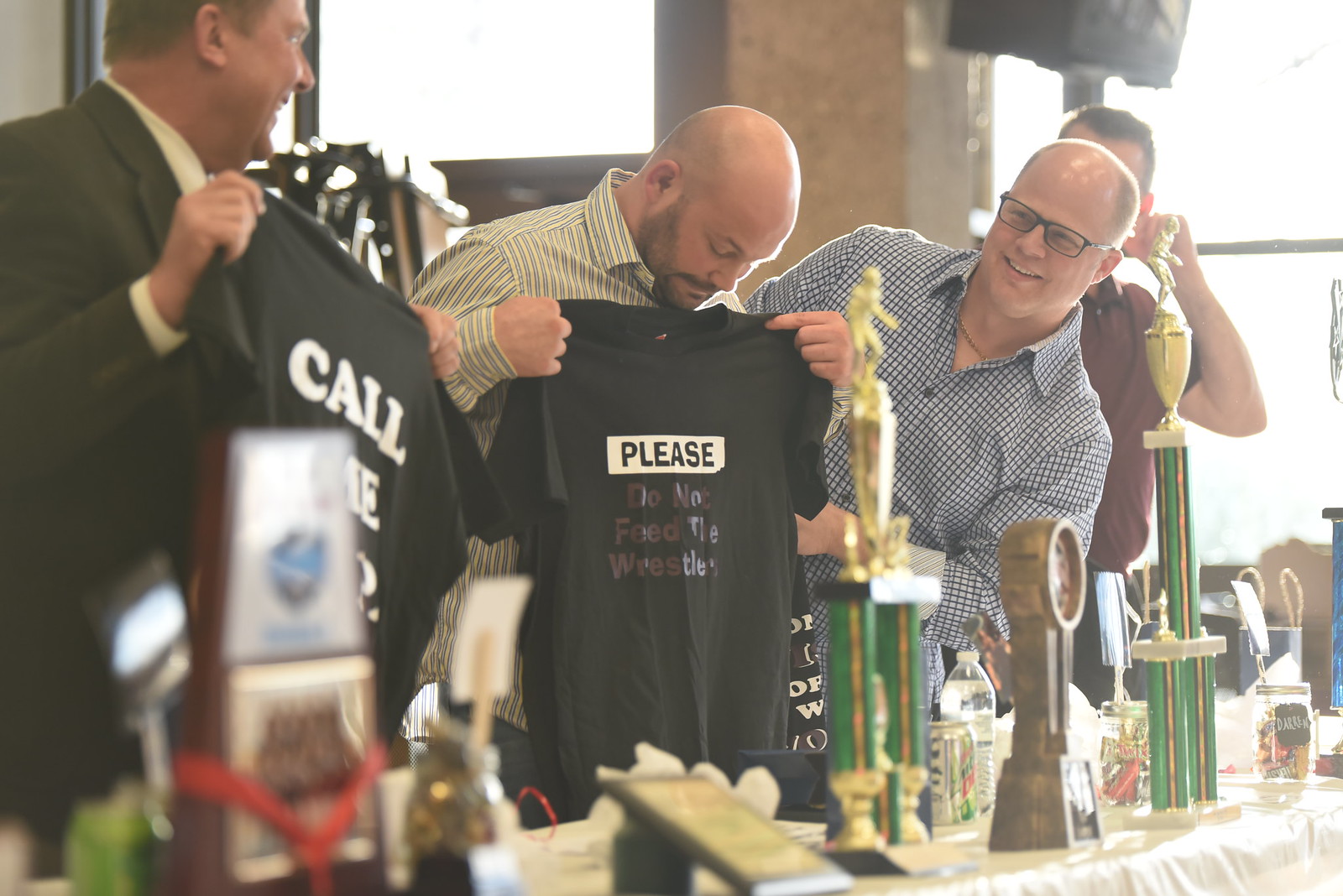The photograph captures an indoor scene bathed in natural light pouring in from the windows behind a group of four men standing behind a table draped in a light gray tablecloth. The table is adorned with multiple green and gold trophies, soda cans, plastic water bottles, and a jar. The image seems to depict a trophy presentation or awards ceremony. 

On the far left, a man dressed in a black suit and a white button-up shirt holds a black short-sleeved t-shirt that reads "Call", with the remaining text obscured by one of the trophies. To his immediate right stands a bald man sporting a striped light green and white button-up long-sleeved shirt, holding a black t-shirt with the slogan "Please do not feed the wrestler," with "Please" highlighted in white. 

Next to them, a man in a blue and white plaid shirt with glasses is seen leaning in and laughing, partially obscuring the fourth man on the far right, who is wearing a red polo shirt and whose face is not visible. The lively interaction and the humorous t-shirts hint at the informal, celebratory nature of the gathering.